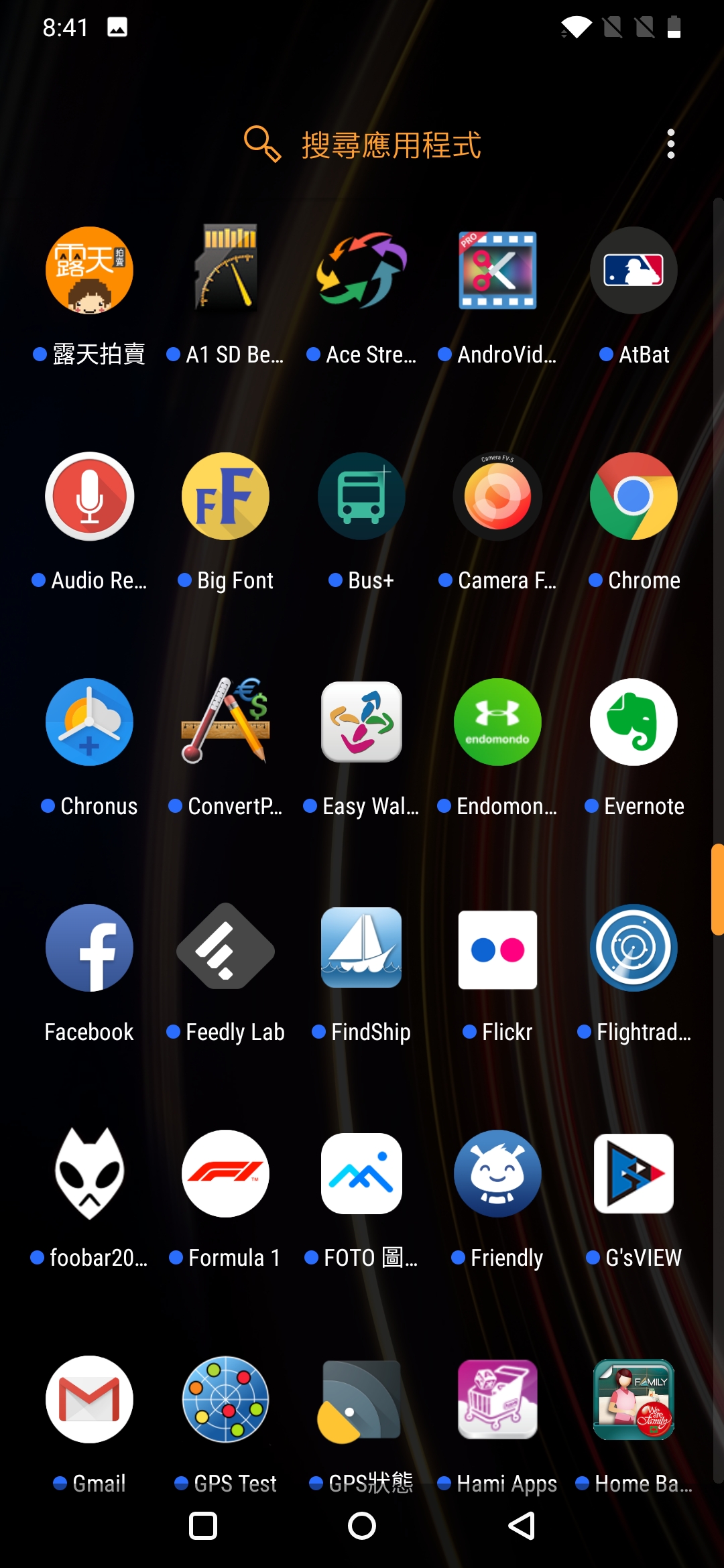The image displays a cell phone screen with a rectangular shape and a pure black background. In the top left corner, the time is displayed as "8:41" adjacent to a white square with a small black segment at the bottom. To its right, there is a fully-filled fan icon followed by several grey icons, each depicted as small boxes with a vertical line descending from the top left to the bottom right. Further right, there is a grey battery icon partially filled with white at the bottom.

Immediately below this, there is a row of characters including an orange magnifying glass icon and text in what appears to be Chinese or an ancient language. Beneath this row, the screen is structured into a grid of icons arranged in six rows and five columns. This grid encompasses applications such as Chrome, At Bat, Audio Recording, BigFont, FindShip, Facebook, Gmail, GPS Test, Homebase, Flightradar, and Flickr. Additionally, some icons are labeled in characters that are not recognizable or readable.

The overall layout and details of the screen indicate a well-populated and organized display featuring a variety of applications, some with specific functions denoted by their names or unreadable characters.